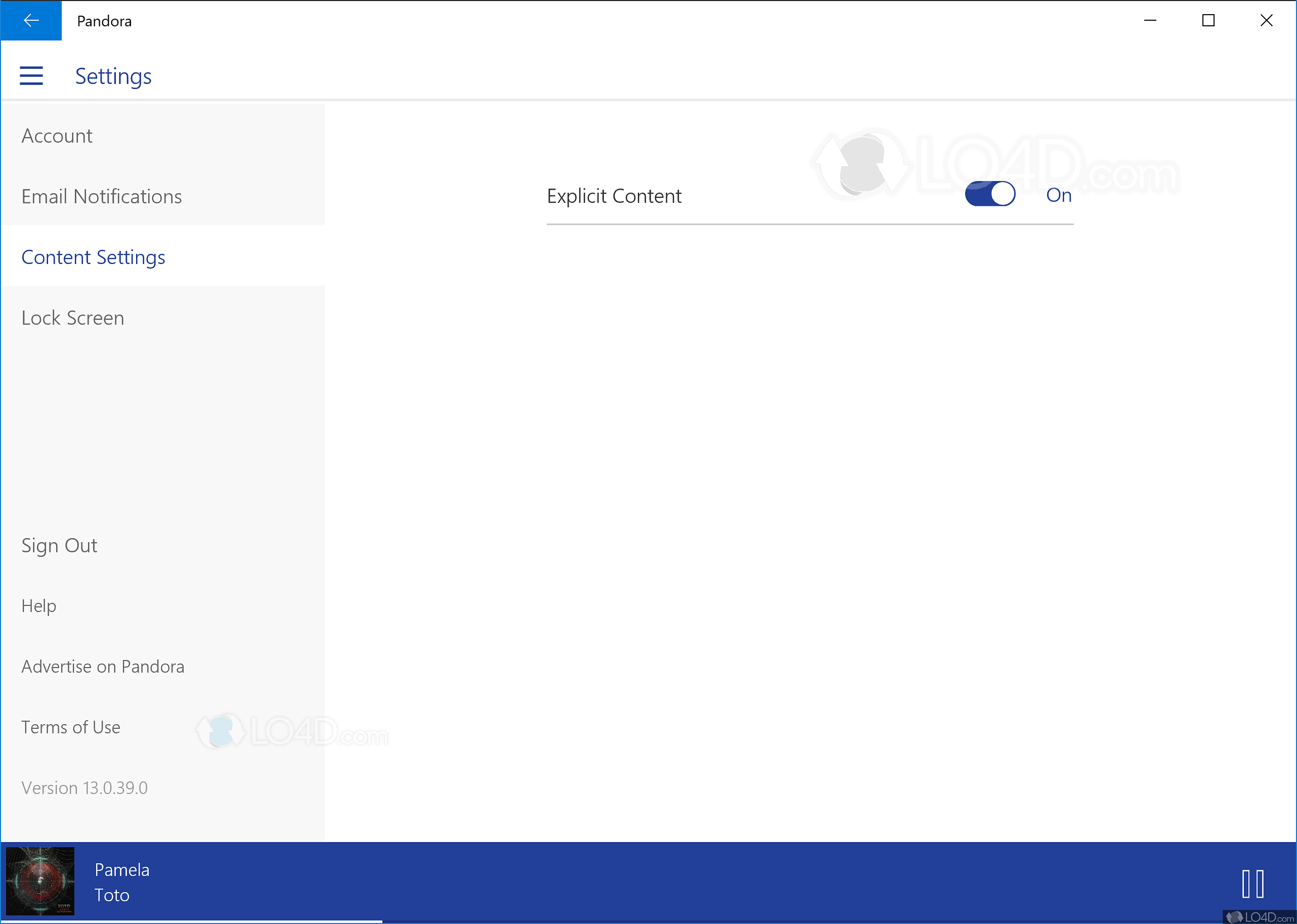The image is a screenshot of a desktop screen displaying the Pandora settings interface. 

The screenshot features a bordered frame where the top border is faint and black, and the side and bottom borders are faint and blue. At the top of the interface, the word "Pandora" is prominently displayed in black ink. Directly below "Pandora," there's a white arrow over a blue background pointing to the left, indicating a back navigation option. Beneath the arrow icon, there are three horizontal lines representing a menu icon, also styled with blue ink. The word "Settings" is written in blue ink next to these lines.

Within the settings menu, several options are listed, including "Accounts," "Email Notifications," "Contact Settings," and "Lock Screen," all in grey ink. "Content Settings" is highlighted in blue ink, indicating that it is the active selection. 

The screen displays the "Content Settings" section, which features a white background. The headlining option in this section is "Explicit Content," next to which there is a toggle switch. This switch is currently set to "On," showing a white circular knob on a blue slider background with the word "On" written in blue next to it.

At the bottom of the screen, a blue band indicates that a song is playing, though the text on the band is partially obscured. It appears to say "Pamela."

Additional options listed at the bottom of the settings interface include "Sign Out," "Help," "Advertise on Pandora," "Terms of Use," and the version information of the application.